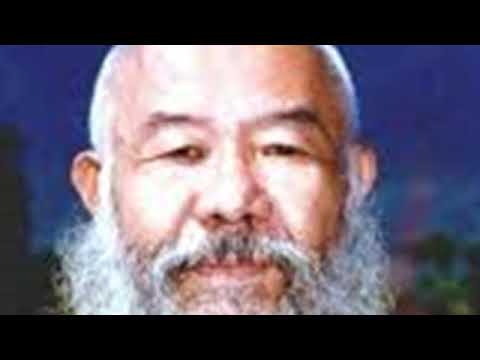The photograph is a close-up of an older man's face, distinctly Asian in appearance, with a serene and slightly serious expression. He has short white hair and a substantial, frizzy beard that is predominantly white with strands of black and gray interspersed throughout. His dark eyebrows contrast with his squinty, droopy eyes that reflect his age. The man’s ears are partially visible, peeking out from behind his long beard. The background consists of a blurred mix of a blue sky and green trees, creating a soft, natural backdrop that makes it difficult to distinguish specific details. The image itself has a slightly pixelated quality with noticeable horizontal black strips at the top and bottom, giving it the appearance of a screenshot from a video. The photograph focuses solely on his face, which is framed in the center, with the top cut off at the mid-forehead and the bottom just above his chin.